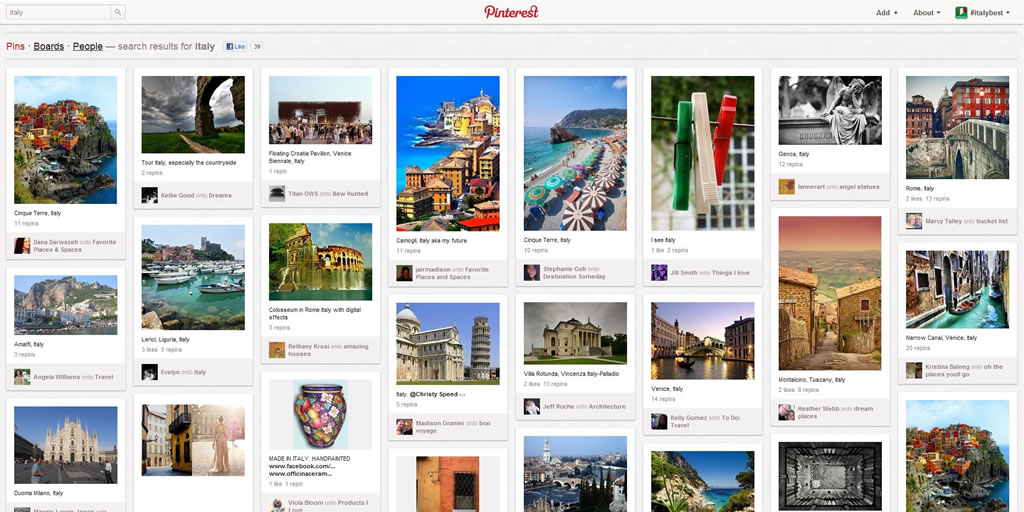This is a detailed desktop screenshot of the Pinterest app featuring search results for "Italy." The background is gray, creating a neutral canvas for the colorful thumbnails. 

At the top left of the screen, there's a small search bar. Centered at the top, you can see the Pinterest logo in red. On the far right, there are sections marked "Ad" and "About" in blue letters, followed by a "Login" button that mimics the Facebook login design.

Below the top menu, the left side of the screen has text that reads "Pins, Boards, People," followed by the phrase "Search results for Italy," indicating the user's search query. The main section of the page is populated by various thumbnail posts that showcase Italian architecture, food, and other cultural items.

Each post follows a consistent format: a large square thumbnail image at the top, a brief description beneath it, and a small thumbnail of the user’s profile picture along with their name or board name. The posts are arranged in vertical rows of three and are evenly distributed down the page. 

In total, there are 24 thumbnails visible on the screen. The top left thumbnail features a stunning image of a city built into the side of a mountain overlooking the ocean, complete with a short description and user information below it. This structured layout continues systematically for all other posts, providing a visually rich exploration of "Italy."